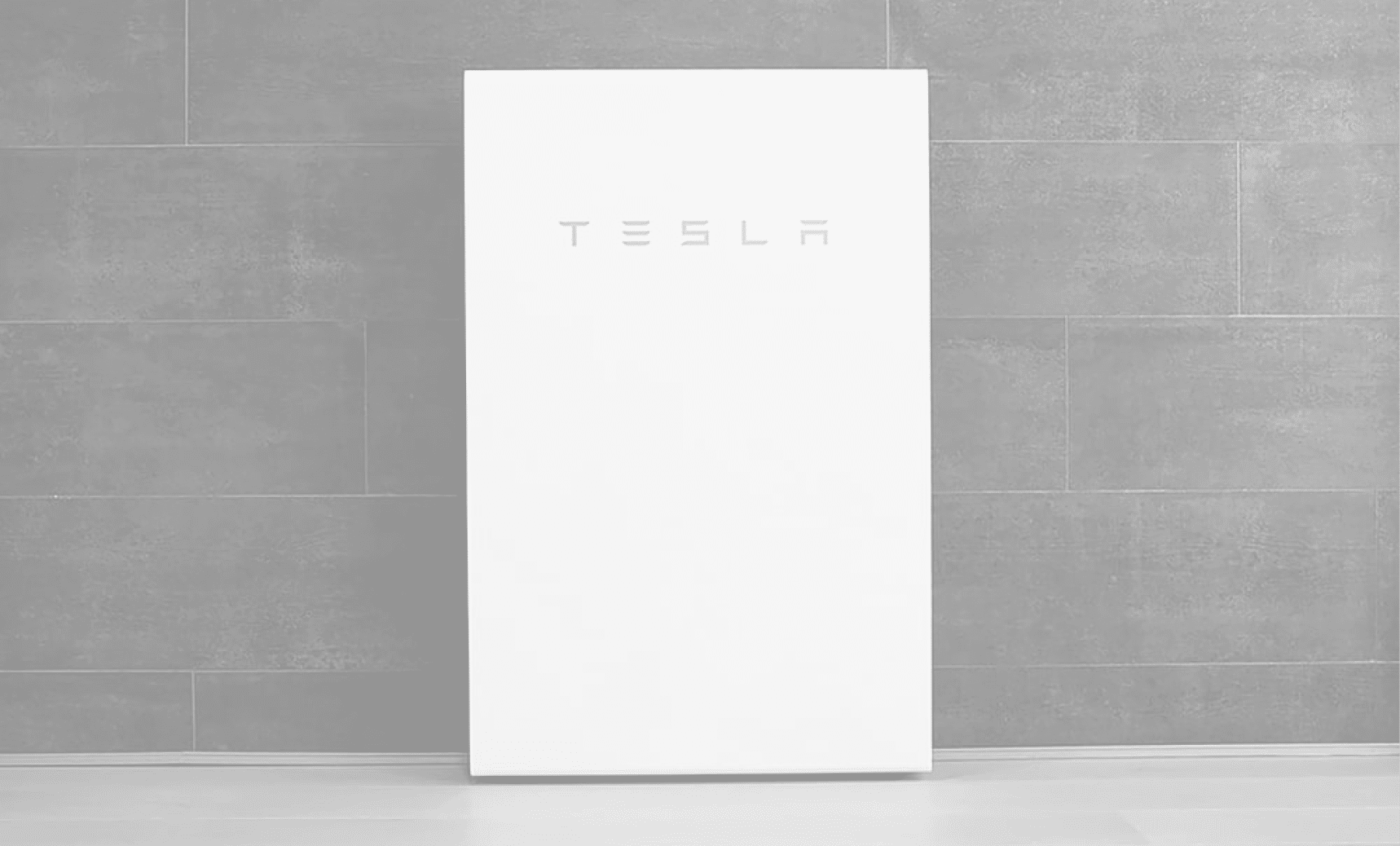A professionally photographed image showcases a minimalistic setting, possibly for an advertising campaign. The image is presented in a horizontal, landscape orientation, providing a broad view of the elements.

The backdrop is composed of large, flat, grayish stone bricks arranged in a neat, orderly fashion. They exhibit a medium shade of gray, and their individual presence is accentuated by fine white lines that separate each brick. The worn, slightly faded texture adds a sense of age and authenticity to the wall.

Transitioning from the wall, the bottom portion of the image features a flat gray surface, possibly serving as a floor or tabletop. This surface merges seamlessly with the wall through a subtle edge, hinting at a clean, continuous design.

Centrally positioned against this minimalist background is a rectangular white box, oriented vertically. This imposing element stands upright on the gray surface, leaning slightly back against the wall. The box prominently displays the brand name "Tesla" in sleek, gray text. Interestingly, the letters "E" and "A" of "Tesla" are unique; their inner sides are open, creating a stylized, modern look that draws attention.

Overall, the composition is striking in its simplicity, highlighting the elegance of the Tesla brand through a clean and subdued aesthetic.